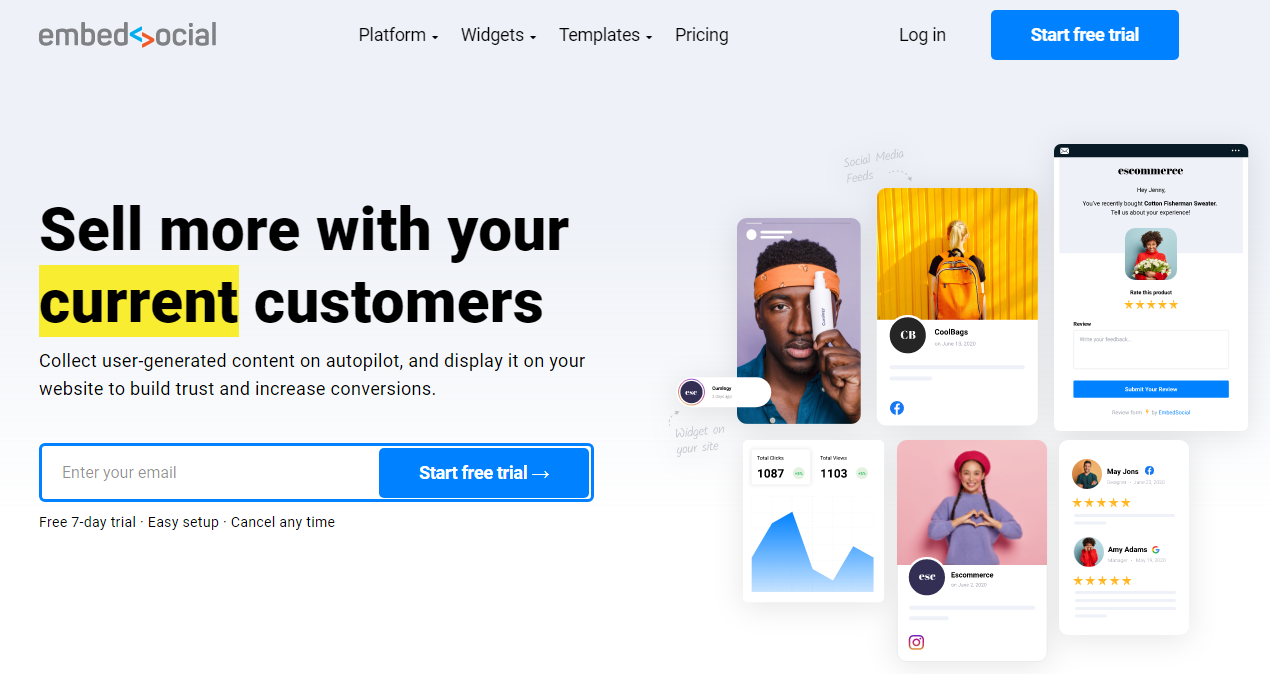Screenshot of the EmbeddedSocial Application Interface

The screenshot captures the user interface of an application named EmbeddedSocial. The top section of the interface features a header labeled "Platform Widgets Template" with an adjacent drop-down menu and pricing information. Towards the right of the header, there is a "Login" option, all set against a light grey background. On the far right-hand side of this header, a prominent "Start Free Trial" button is displayed in white text on a blue rectangle.

Below the header, the left-hand side contains a marketing message: "Sell More with your Current Customers," with the word 'Current' highlighted in a yellow box. This message is followed by a subheading: "Collect user-generated content on autopilot and display it on your website to build trust and increase conversions." An input field accompanied by a blue button invites users to "Enter Your Email" and "Start Free Trial." Beneath this is additional text offering, "Free 7-Day Trial, Easy Setup, Cancel Any Time."

To the right, there is a visual display of various user-generated content examples. The first image shows a dark-skinned man holding up a bottle of skincare product. The second image features an individual displaying an orange backpack against a yellow background. This is followed by a series of diverse content, including a picture captioned "Commerce," an image of someone leaving a rating, some data charts, a person forming a heart shape with their hands while smiling at the camera, resembling an influencer, and two more review snapshots.